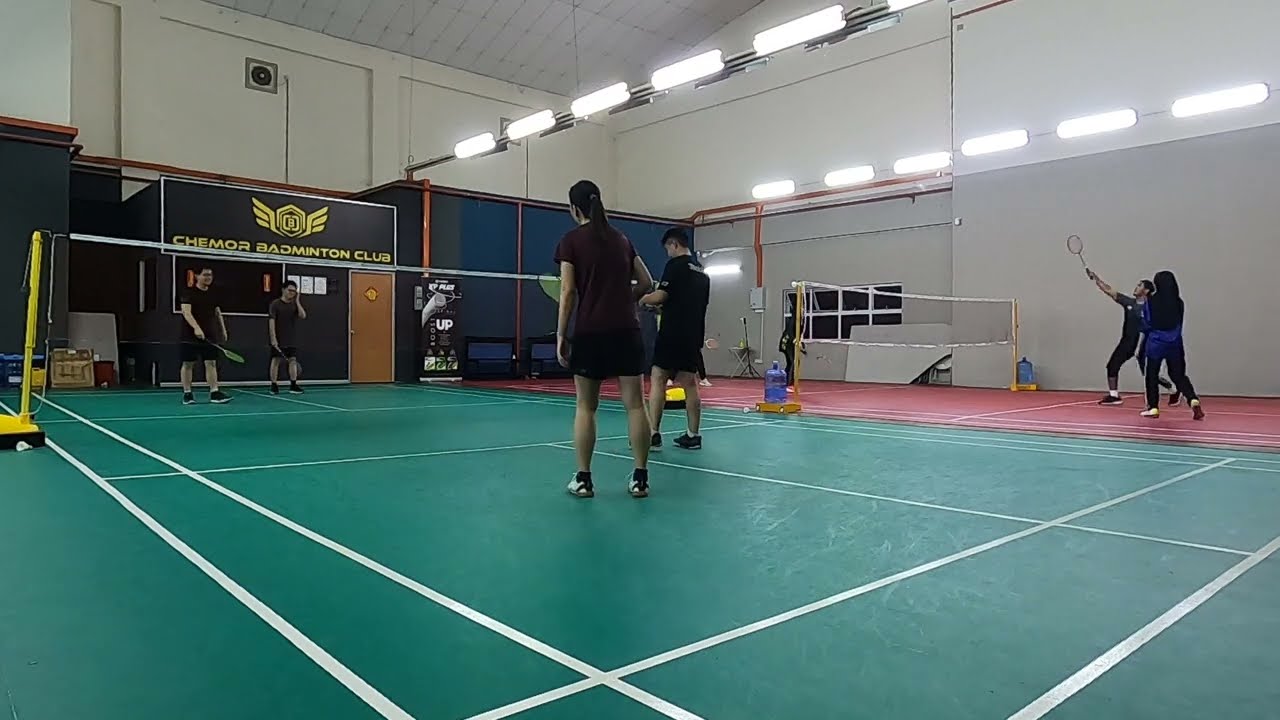This detailed image captures an indoor badminton club with two adjacent courts. The gymnasium features white walls topped with gray along the bottom, and a window on one side of the building. White panels form the roof, complemented by fluorescent lights hanging halfway down the spacious room. In the foreground, the green badminton court, marked with crisp white lines, hosts four players: a female with her hair in a ponytail wearing a burgundy shirt, black shorts, and white shoes stands at the center, alongside a man in a black shirt and white shorts. The red or tan court in the background is similarly marked with white lines and is currently occupied by two visible players, both on the same side of the net. Each court has two posts supporting a black and white net. The back wall displays the lettering “Shamor Badminton Club”.